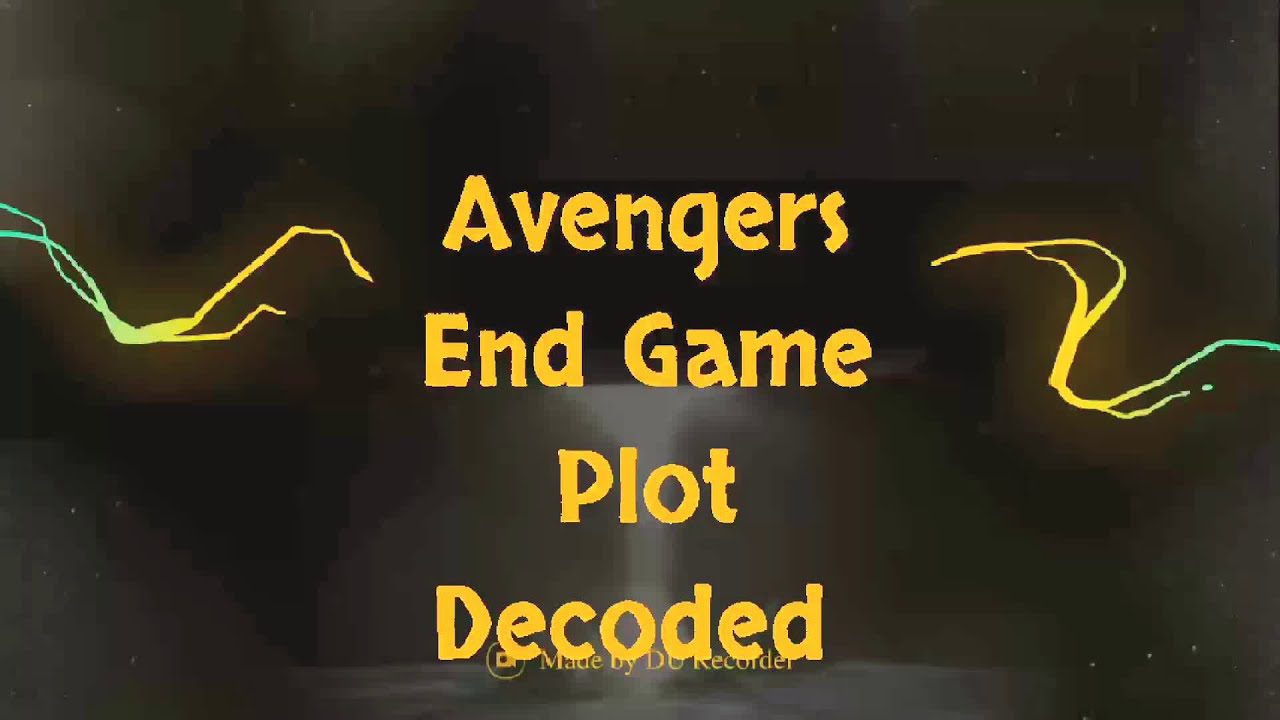The screenshot features a visually simplistic and somewhat primitive graphic design. Set against a predominantly black, smoky background, the centerpiece consists of four lines of large, yellow text that reads: "Avengers," "Endgame," "Plot," and "Decoded." Surrounding this central text are dynamic, squiggly lines or streaks that start close to the text in yellow and gradually fade into green before disappearing off the edges of the image. Beneath the primary text, in smaller yellow letters, a byline states that it's "Made by DC Recorder," though partially obscured by the word "Decoded." These yellow and teal elements create an impression of electricity or digital swirls converging from the sides towards the center, reinforcing the dramatic theme of the graphic.